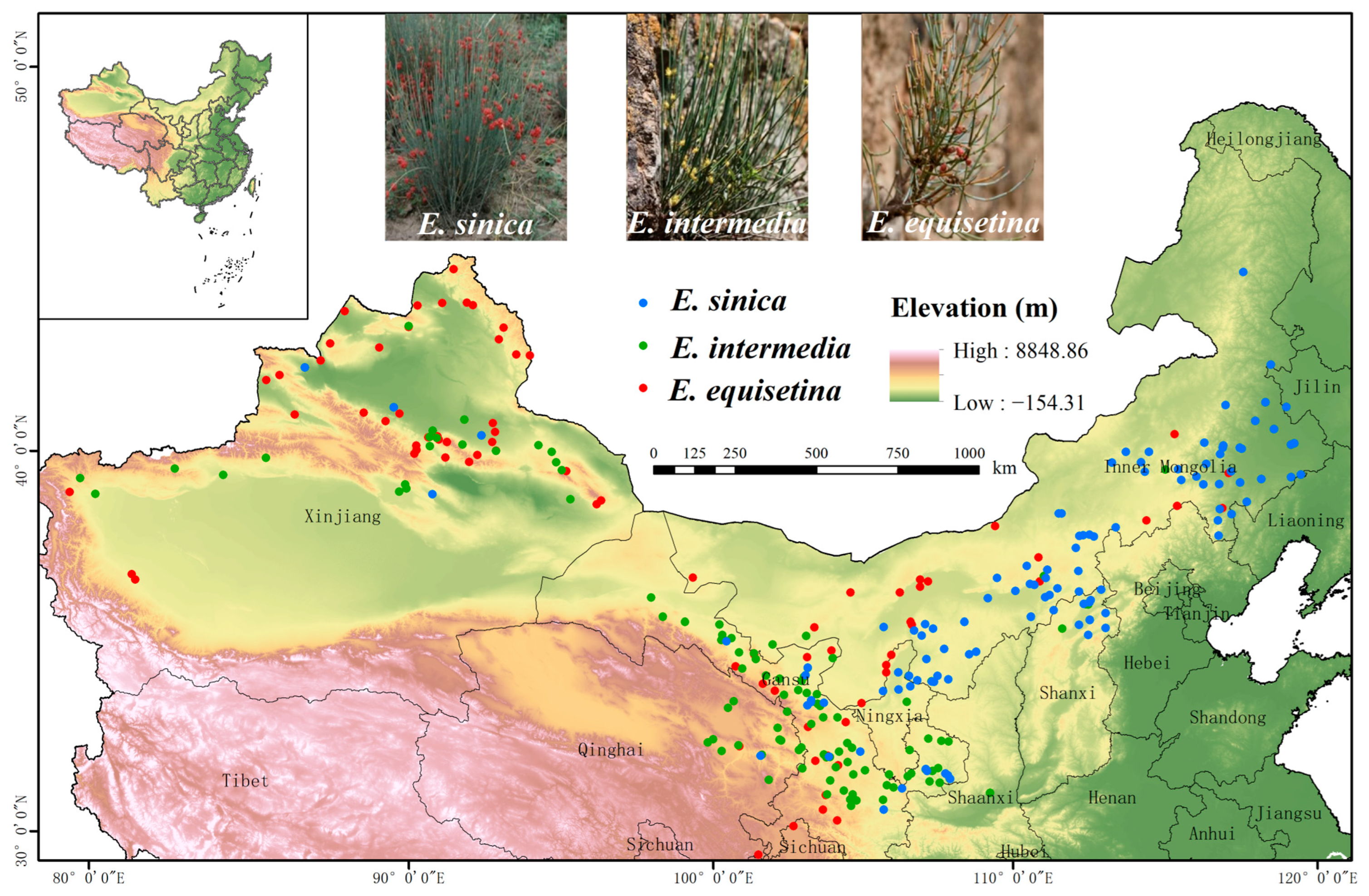The image is a detailed topographical map primarily depicting China and possibly extending to other parts of Asia. This map is characterized by a watercolor-like background with shades of green, tan, and pink, along with precise black ink lines for geographical details. Scattered across the map are red, blue, and green dots which correspond to the locations of three plant species: E. senecia (blue dots), E. intermedia (green dots), and E. esquinetina (red dots). A key situated in the middle of the page identifies these species and their respective dot colors.

At the top of the map, there are three photographs showing what each plant looks like in real life: E. senecia with red flowers, E. intermedia with tiny yellow flowers, and E. esquinetina with red flowers and sparse green branches. Additionally, there is a larger inset map of China in the upper left corner highlighting the concentration of these plants. The elevation is indicated by a color chart, revealing the terrain's high and low points, which further correlates with the plant distribution. The map also includes place names written in Chinese, with notable regions such as Tibet and its mountainous areas marked in red.